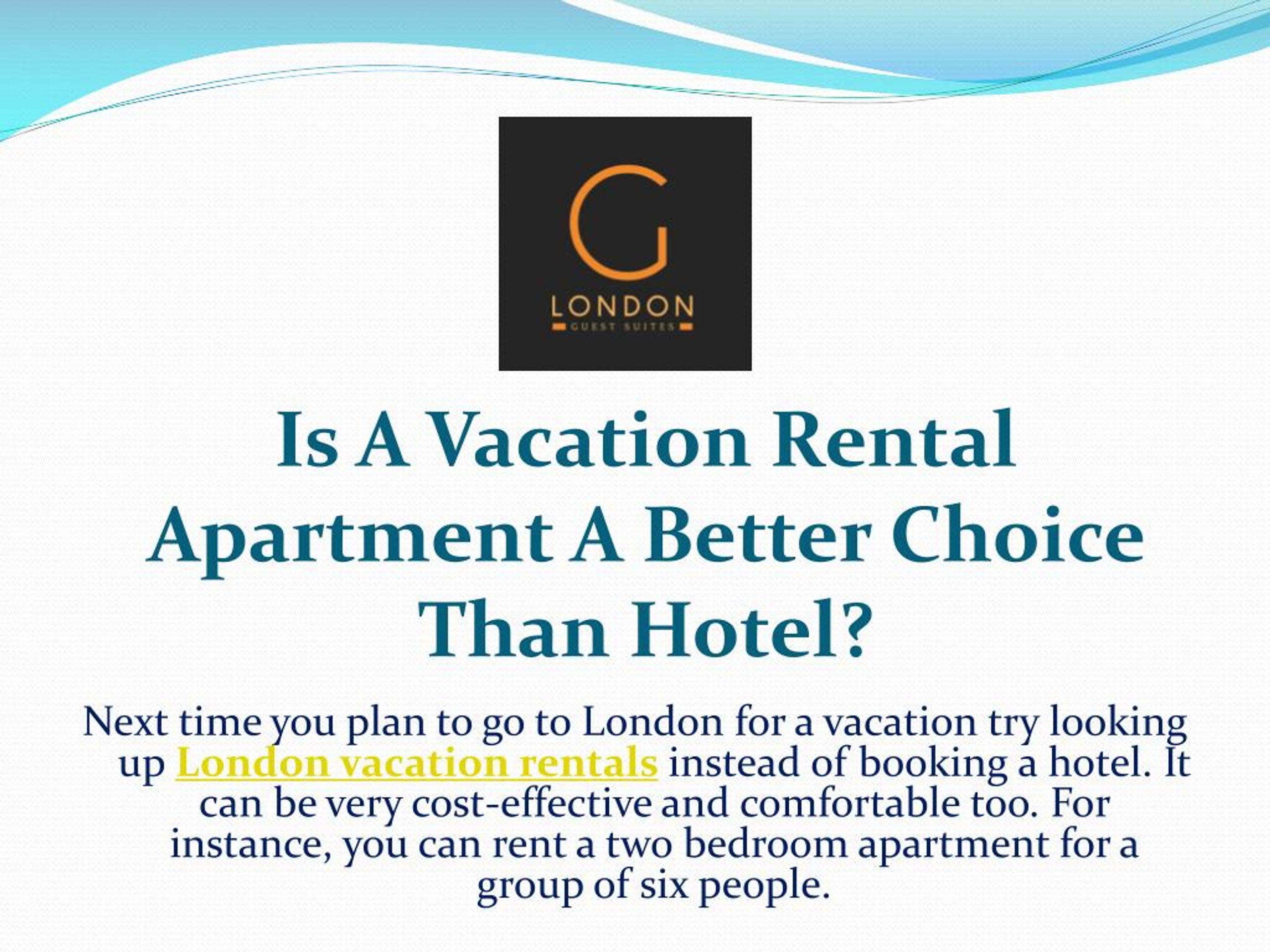The advertisement promotes vacation rental apartments as a superior alternative to traditional hotels or motels for travelers visiting London. At the center of the image, there is a question highlighted in blue: "Is a vacation rental apartment a better choice than a hotel for your next trip?" Above this, in a black box, is a neon "G" logo with the words "4G London Guest Suites" beneath it, indicating the brand being advertised. The background is predominantly white, decorated at the top with blue wavy lines interspersed with white stripes. Below the central question, the ad encourages travelers to consider London vacation rentals, with the text "London vacation rentals" emphasized in yellow, suggesting they can be cost-effective and comfortable. It even highlights the example of renting a two-bedroom apartment for a group of six people as an economical and convenient option. The ad implies a clickable hyperlink, though it can't be interacted with in this format. Overall, the advertisement is a persuasive effort by 4G London Guest Suites to shift potential vacationers' preferences from traditional hotels to vacation rental apartments.